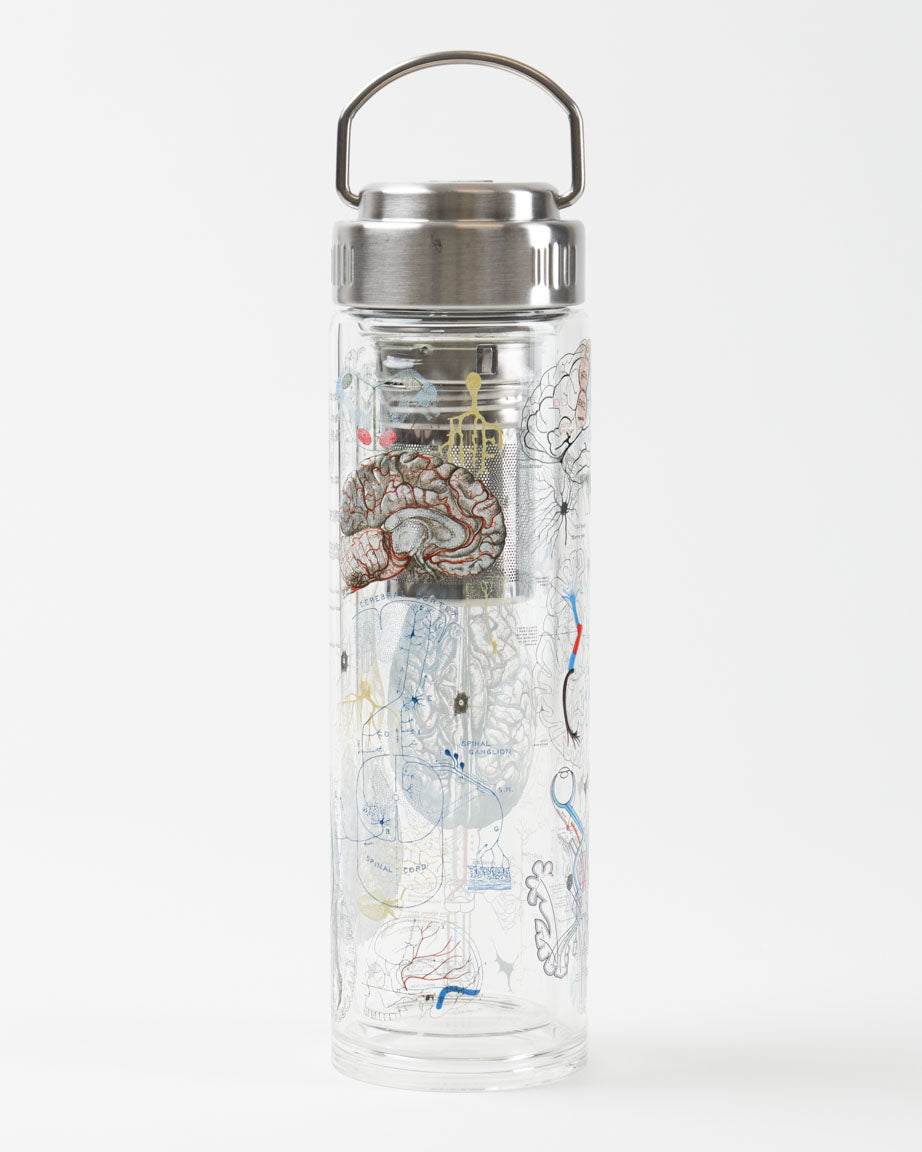The image is a professionally edited product photograph of a reusable glass water bottle, set against a solid white background typically used for commercial purposes such as online shops or catalogs. The rectangular image features a cylindrical, clear glass bottle with a large, screw-on, metallic cap that resembles sterling silver. Attached to the cap is a small perforated cylindrical filter and a carrying handle positioned upright for convenience. The surface of the bottle is adorned with detailed anatomical diagrams, particularly of the human brain and nervous system, featuring multiple intricate illustrations. Despite the clear nature of the glass, there are no physical objects inside the bottle, only the detailed drawings that encase it, contributing to a scientific, clinical aesthetic.